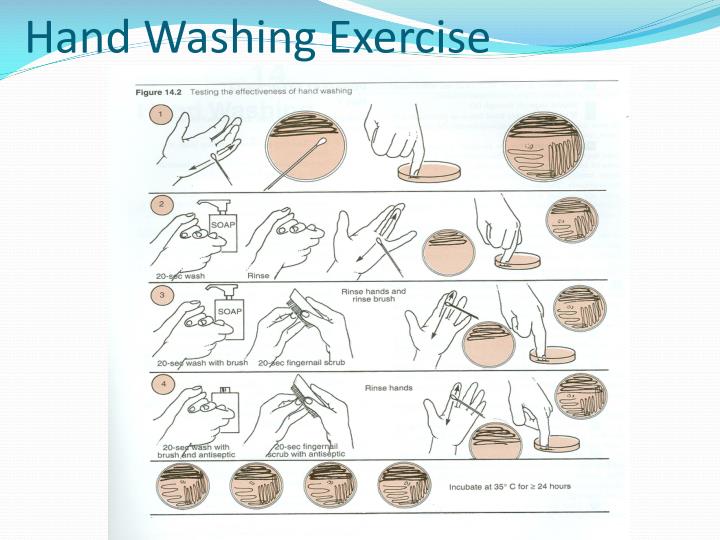A detailed illustration of a hand-washing exercise is depicted, labeled "hand-washing exercise" in blue print against a light blue and white wavy background. Below, it reads "Figure 14.2: Testing the Effectiveness of Hand-Washing." The exercise consists of four rows, each describing a different hand-washing method and its subsequent bacterial testing process using Petri dishes. 

In Row 1, a hand is simply swabbed and the swab is placed into a Petri dish, showing various bacteria as squiggly lines. 

Row 2 illustrates a 20-second hand wash with soap, followed by rinsing. The hand is then swabbed and the swab is placed in a Petri dish.

Row 3 details a 20-second wash with soap and a brush, including a 20-second fingernail scrub. After rinsing both hands and the brush, a swab is taken and placed into a Petri dish.

Row 4 shows a 20-second wash with soap, a brush, and antiseptic, coupled with a 20-second fingernail scrub with antiseptic. The hands are rinsed, swabbed, and the swab is then placed into a Petri dish. 

Finally, the text instructs that all Petri dishes should be incubated at 35 degrees Celsius for 24 hours to observe bacterial growth. The overall illustration provides a comparative analysis of bacterial presence in each Petri dish, highlighting the effectiveness of different hand-washing techniques.